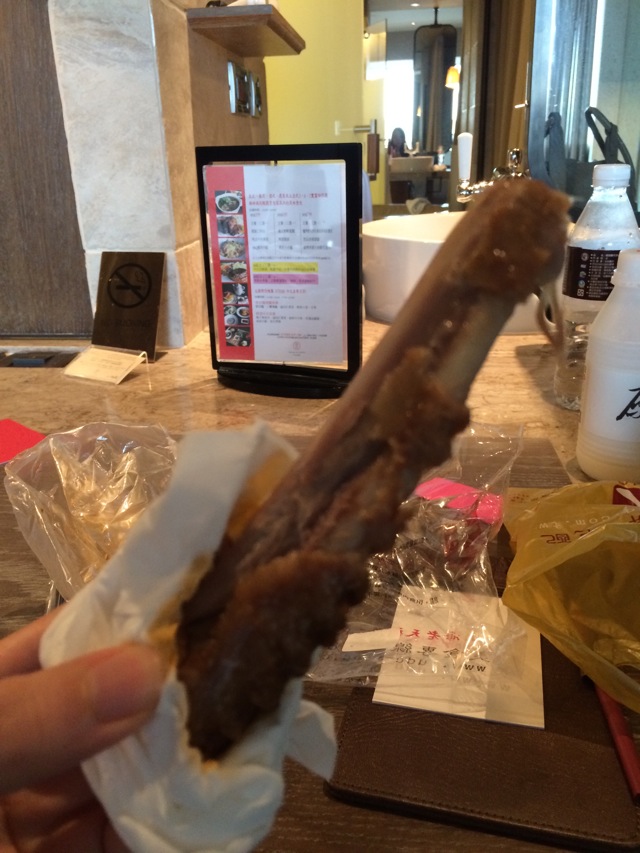A photograph captures a scene likely set in a restaurant or kitchen environment. Central to the image is a large piece of meat, possibly a rib or another barbecued or deep-fried item, held by a woman's thumb and forefinger. The meat is wrapped in a white paper towel or napkin. On the countertop in the background, there is a distinct Asian food packaging with visible labeling, suggesting the meat may be part of an Asian dish. Also visible are remnants of plastic packaging, other plastic bags, and a water bottle. A black-framed menu or recipe display, featuring various dishes and text, stands prominently on the table. Additionally, a white bowl is situated nearby. In the mirror at the end of the hallway, the reflection of the photographer is faintly visible, adding depth to the composition. The backdrop includes a large window, a cabinet, lighting fixtures, and hints of a table with chairs, reinforcing the indoor setting.